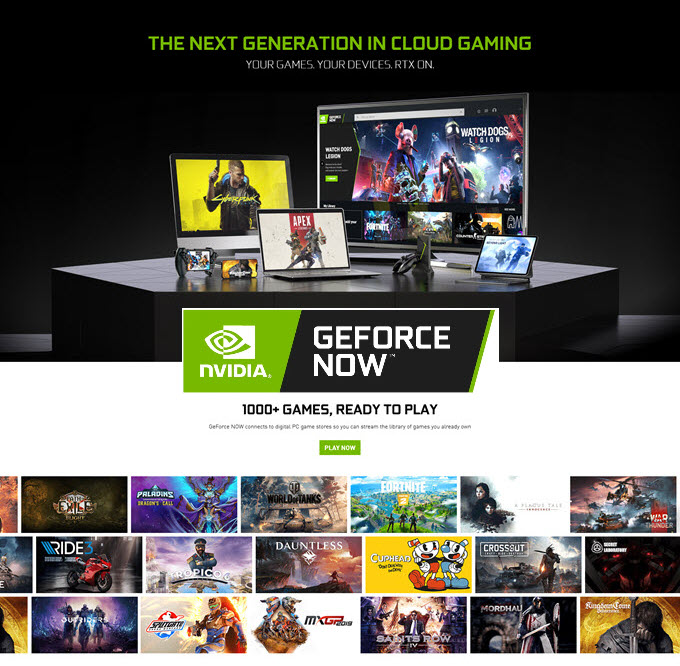**Caption:**

"Introducing the next generation in cloud gaming with NVIDIA GeForce Now — your games, your devices. The advertisement showcases a sleek lineup of a TV, desktop, laptop, tablet, and cell phone, each displaying the latest gaming titles like Apex Legends and Watch Dogs. A game controller is prominently featured, symbolizing seamless gameplay across various platforms. With access to over a thousand games, this cloud gaming service offers a diverse library including Ride 3, Dauntless, Crossout, Fortnite, Path of Exile, Saints Row, and Mordhau, among many others. Experience the future of gaming with NVIDIA GeForce Now."